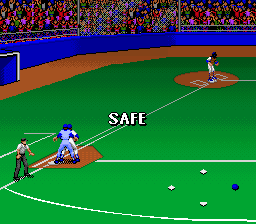This screenshot captures a moment from a video game depicting a baseball scene. The image highlights a batter who has successfully reached first base, indicated by the word "Safe" on the screen. Visible elements include home base and third base, while the second base remains out of the frame. In the bottom right corner, there is a graphical representation of the bases arranged in a diamond pattern, corresponding to home, first, second, and third bases. Notably, the first base icon is colored blue, suggesting that a player is currently occupying it, while the other bases are marked with white icons, indicating they are empty.